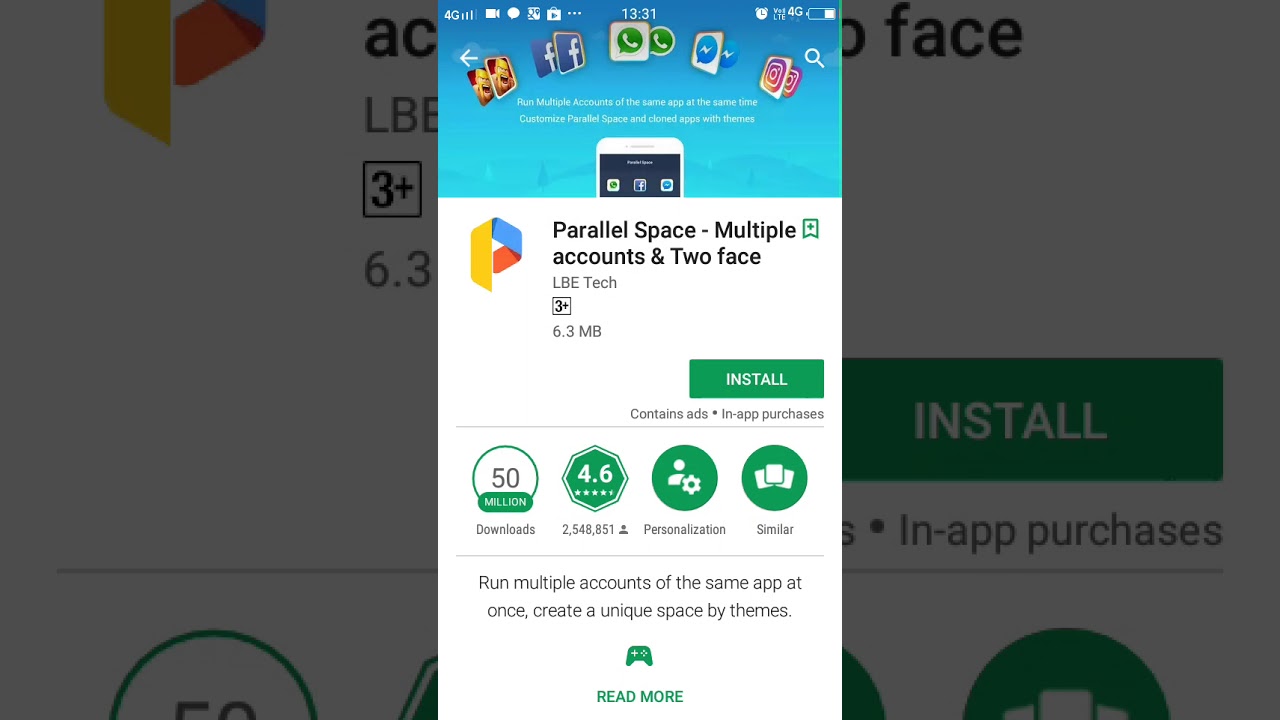The image depicts a narrow screen interface with a white background and a blue top section. The interface features numerous green buttons and headings, alongside an installation button. The prominent heading on the screen reads "Parallel Space: Multiple Accounts Plus," indicating the app's purpose of managing multiple accounts. A slightly obscured text below hints at "Accounts and Two Face," which suggests functionalities related to dual account management.

At the top of the page, there are multiple headings possibly representing various media sites, including recognizable icons such as Facebook, and another with a white zigzag on a blue background, among others that are less identifiable. The screen also contains descriptive text promoting the app, stating, "Run multiple accounts of the same app at once" and "Create a unique space by themes." Users are prompted to read more for additional details before deciding to install the application.